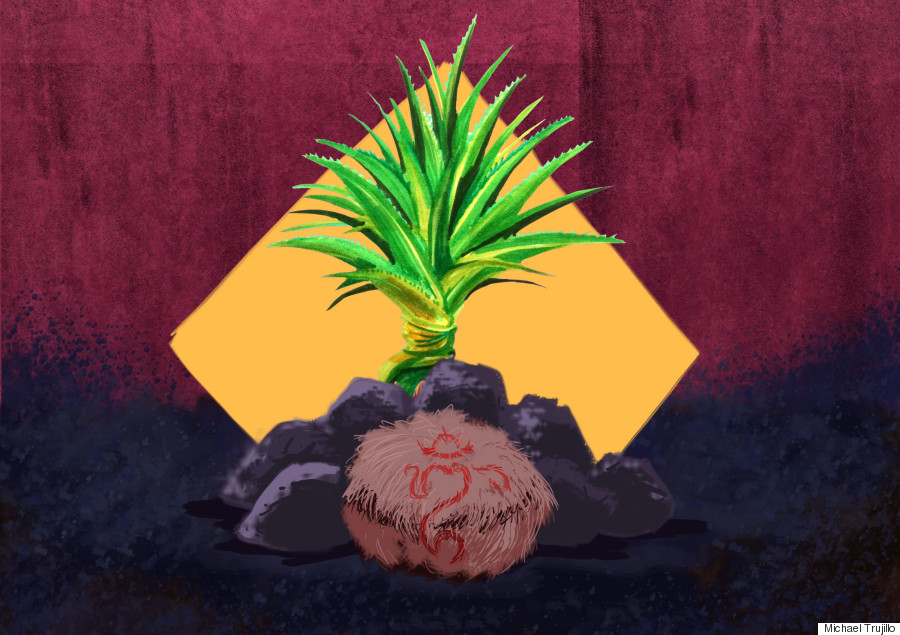The image is an artwork by Michael Trujillo featuring a vibrant scene with multiple elements. In the foreground, there's a green succulent or air plant, reminiscent of an aloe vera or cactus, perched atop a pile of about ten dark gray rocks. Beside this plant is a small, pink, fluffy furball bearing an intricate red symbol or markings. Behind the green plant, a square piece of orange-yellow paper or cardboard adds a contrasting geometric element. The background exhibits a gradient of dark purple and maroon hues, blending seamlessly into darker shades. The bottom right corner of the image includes a watermark, stating "Michael Trujillo" in black text within a small white box. The composition of the painting creates a striking balance of colors and textures, making it visually intriguing.